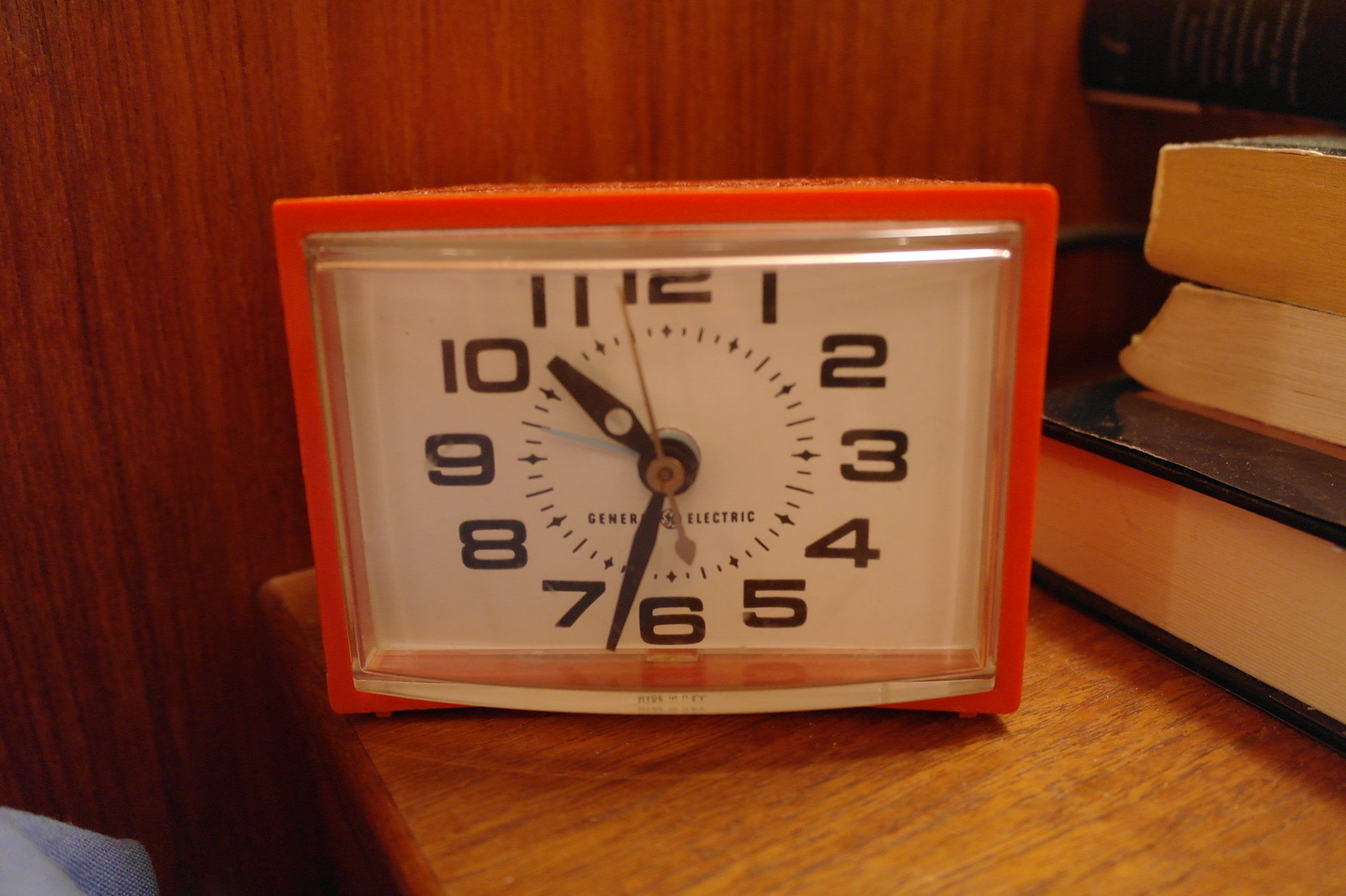This color photograph features a plastic rectangular clock with a distinctive orange trim, prominently displayed on a wooden nightstand. The clock face, which reads 10:32, is white with black numbers ranging from 1 to 12, and includes black hour and minute hands accompanied by a brass-colored second hand. The clock's face also bears the logo "General Electric." Positioned alongside the clock are three stacked books, the bottom one being a hardback. In the background, wooden paneling is visible on the walls, and a blue piece of clothing can be seen in the very left-hand corner of the image, hinting that this scene might be set in a bedroom.